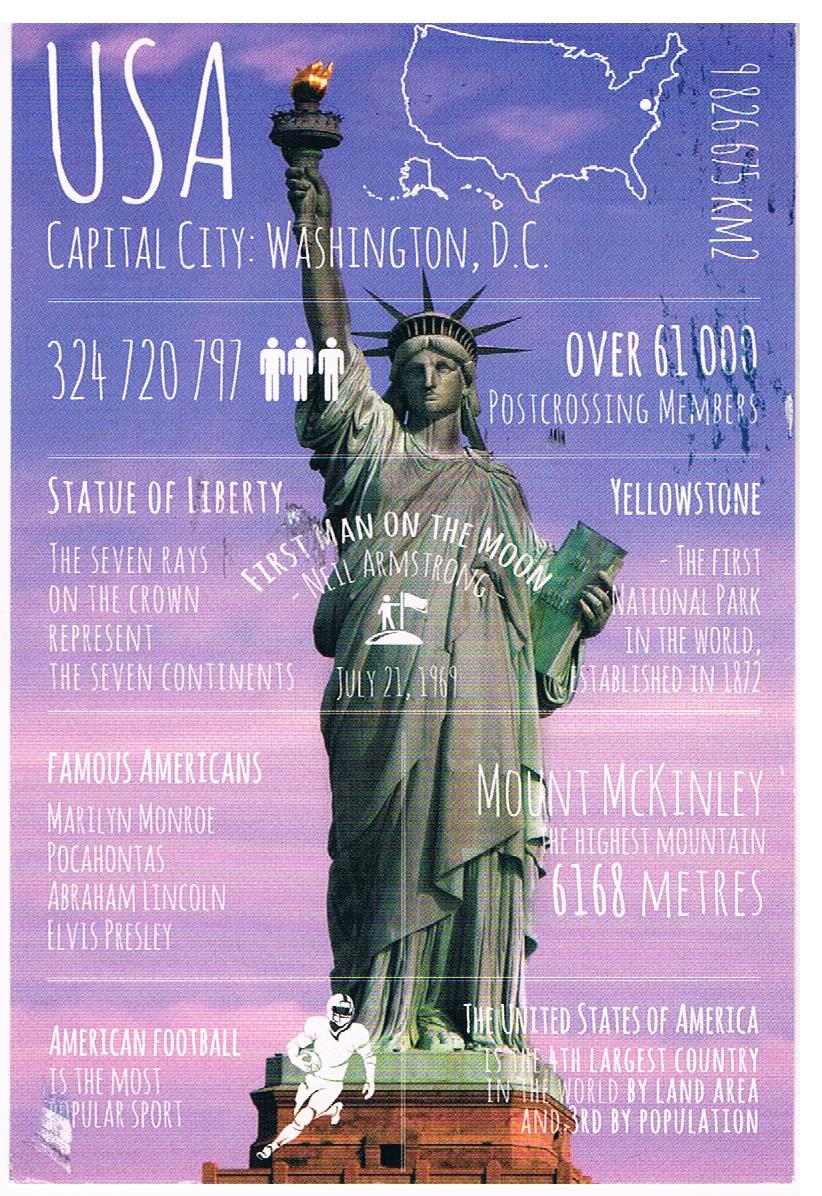This infographic features the Statue of Liberty against a sky that transitions from pinkish tones at the bottom to blue at the top, giving it a photoshopped effect. Superimposed on this background are various pieces of information presented in white, handwriting-like font. 

At the top left, "USA" is written, with "Capital City, Washington D.C." beneath it in smaller text. An outline map of the United States is displayed at the top right, indicating the land area as 9,826,675 kilometers squared. Below this, population data is presented, showing 324,720,797 people, along with a note about over 61,000 post-crossing members.

Details about the Statue of Liberty mention that the seven rays on the crown represent the seven continents. Additional historical and cultural facts are included, such as Neil Armstrong becoming the first man on the moon on July 21, 1969, and Yellowstone being the first national park in the world, established in 1872.

The infographic also lists famous Americans like Marilyn Monroe, Pocahontas, Abraham Lincoln, and Elvis Presley. Mount McKinley is noted as the highest mountain at 6,168 meters. American football is highlighted as the most popular sport, indicated by a white graphic of a football player superimposed above the base of the Statue of Liberty. Lastly, it states that the United States is the fourth largest country by land area and the third most populous.